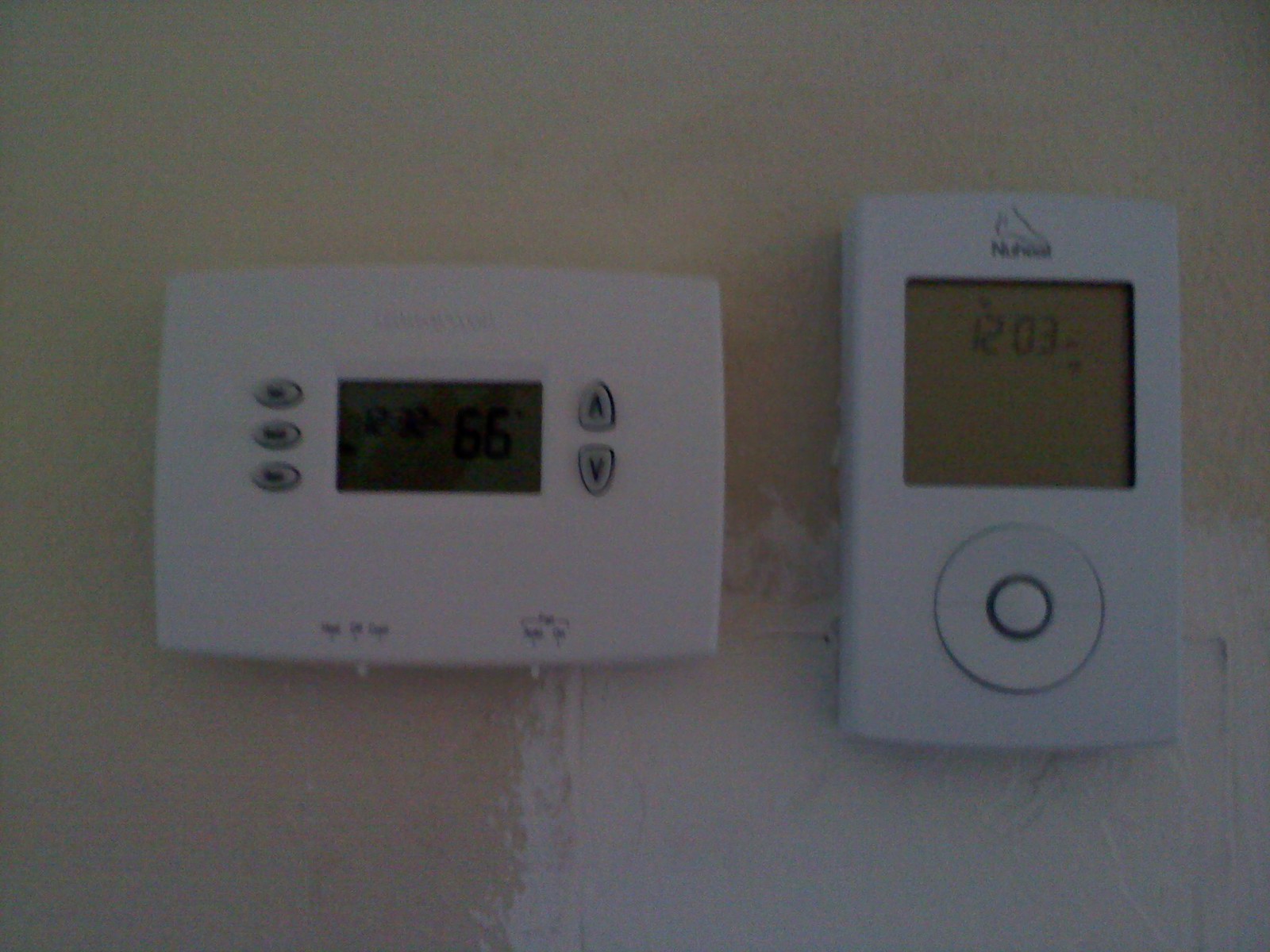The image features an off-white background with predominantly dark and shadow-filled elements, lacking significant illumination. In the bottom right corner, there's a white square with rough edges. Two thermostats are prominently displayed. 

The thermostat on the left features a gray display that is difficult to read due to dim lettering. It has three vertically aligned buttons on the left side and two additional buttons on the right side, one for increasing and one for decreasing settings. Below it, a switch is visible, potentially for toggling settings, though its exact function is unclear.

The thermostat on the right appears to have a logo resembling an "8 foot" symbol and text that partially reads "NU something." Its gray display shows the time "12:03." Below the display, a large circular button is present, characterized by a half-circle design on the top and bottom, with a white circle in the middle intended for pressing.

Overall, the image captures the intricate details of the thermostats against a subdued background, emphasizing their functional features.